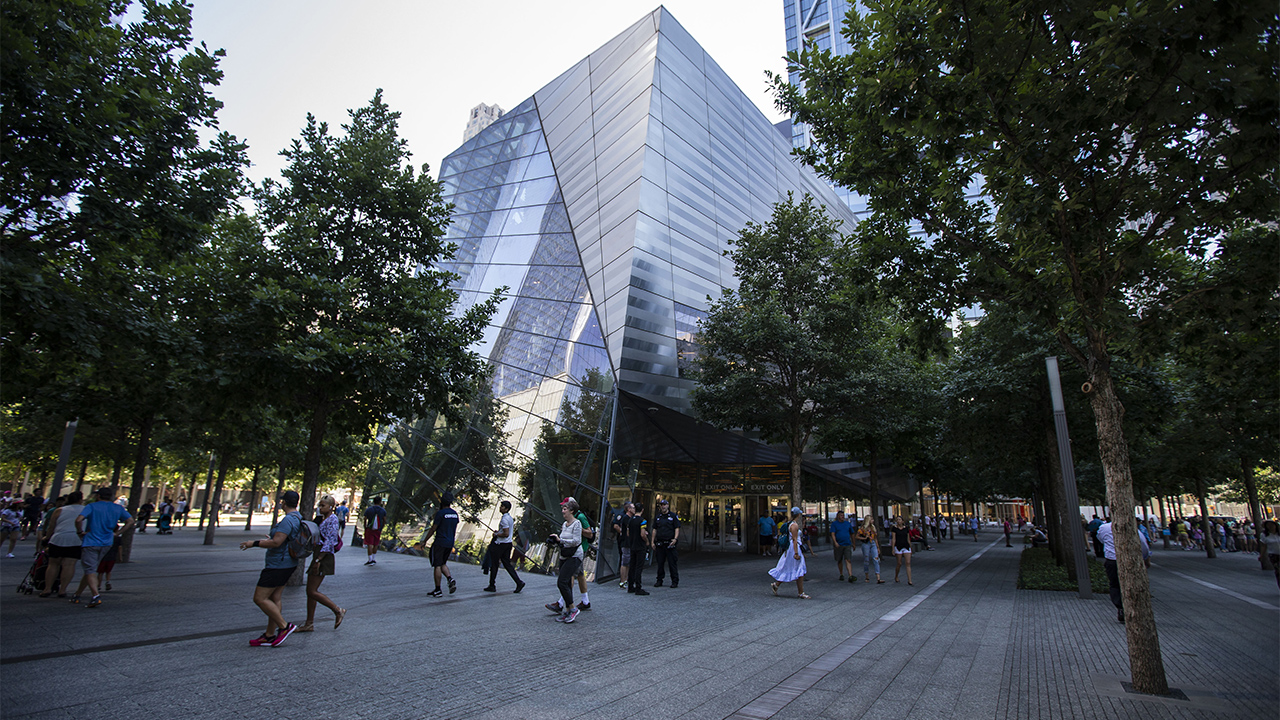This photograph captures a bustling urban scene centered around a distinctive, highly reflective building, likely a community center or public facility. The structure is a four to five-story rectangular edifice, characterized by its mostly glass facade which mirrors the surrounding environment. Notable architectural features include sharp, diagonal window panes and a rectangular window streak that alternates between glossy and bluish matte finishes. The building’s upper section comprises a juxtaposition of mirrored and opaque glass, forming an upside-down right triangular prism effect. 

The ground level of the building is recessed, providing a shaded entryway beneath a large awning, where several police officers or security guards are standing watch. The area surrounding the building is a gray brick-paved courtyard, devoid of roads or cars and bustling with numerous people in summer attire such as shorts and skirts.

The space is well adorned with verdant trees planted in boxed-off areas within the pavement, contributing to a green and lively atmosphere despite the urban setting. The scene is set under a bright, cloudless sky, with sunlight illuminating the spotless, glassy surface of the building and the greenery around. Though closely focused on this main building, the image also hints at other skyscrapers reflected in the glass and a taller building peeking from the background.